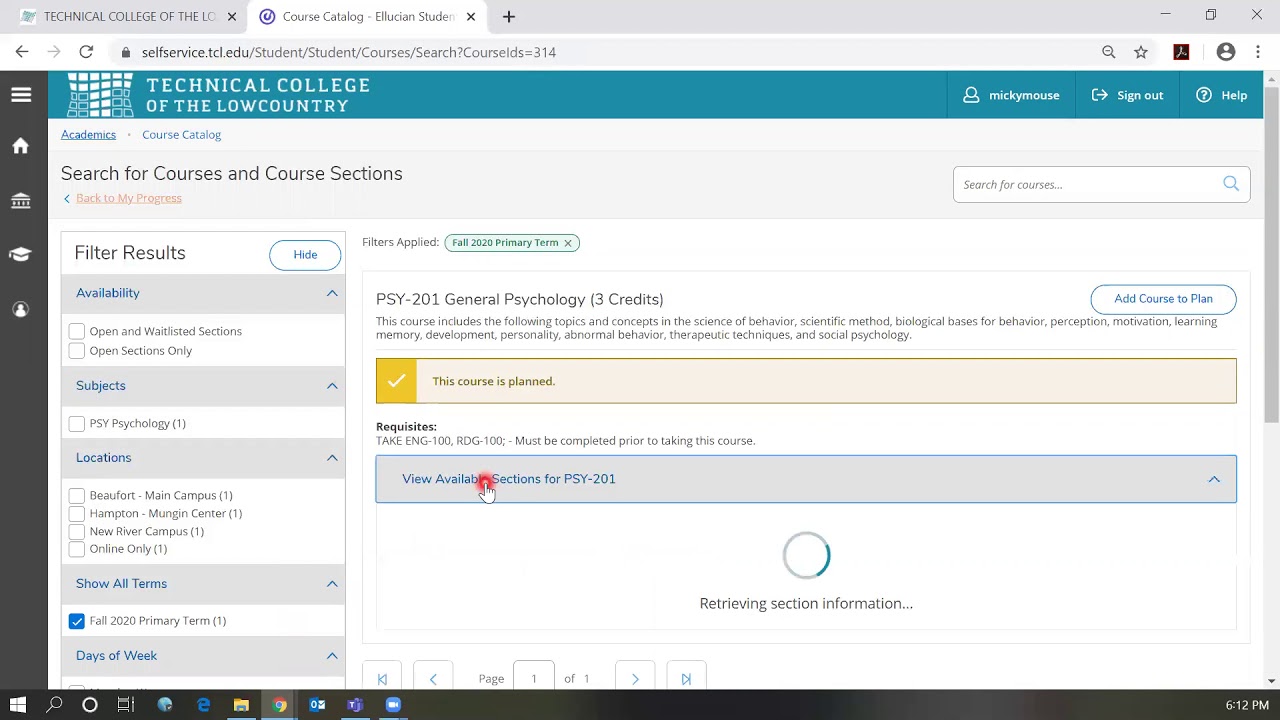This is a detailed landscape-oriented PC screenshot of a website displayed in a browser. The URL in the address bar reads: selfservice.tcl.edu/student/student/courses/search?courseID=314. The tab displaying this page is labeled "Course Catalogue - Ulysses Student," but the title is cut off. Next to it, another tab reads "Technical College of the." Both tabs are set against a light gray background.

Positioned below the URL bar, a blue navigation bar spans the top of the webpage. On the left of this bar, white text reads "Technical College of the Lowcountry," accompanied by a logo comprised of several small white and blue squares. To the right, three white text links are labeled "Profile (Mickey Mouse)," "Sign Out," and "Help."

The main content of the webpage features an off-white background. At the top, bold black text reads "Search for Courses and Course Sections." Directly beneath, there is an orange hyperlink labeled "Back to My Progress."

The left side of the page includes various filters for refining search results, each with a blue title and gray checkbox options. The filters listed are "Availability," "Subjects," "Locations," and "Show All Terms," with "Show All Terms – Fall 2020 Primary Term (1)" already ticked.

The right side of the page displays the search results. The first result is "PSY 201 - General Psychology (3 Credits)" in bold black text, followed by a brief two-line description. Below, a light yellow box with a black check mark contains the text, "This course is planned."

Further down, there is a requisites section with the title "Requisites" in bold black text. It states that "ENGLISH 100" and "RPOG 100" must be completed prior to enrolling in "PSY 201." Below this section, a light gray box with a blue border contains the text "View Available Sections for PSY 201" in blue text. This option has been selected, as indicated by a red circle around the cursor. Below, a loading bar is present with the text "Retrieving section information" in gray.

The bottom of the screenshot displays the standard Windows taskbar, showing the current time as 6:12 PM.